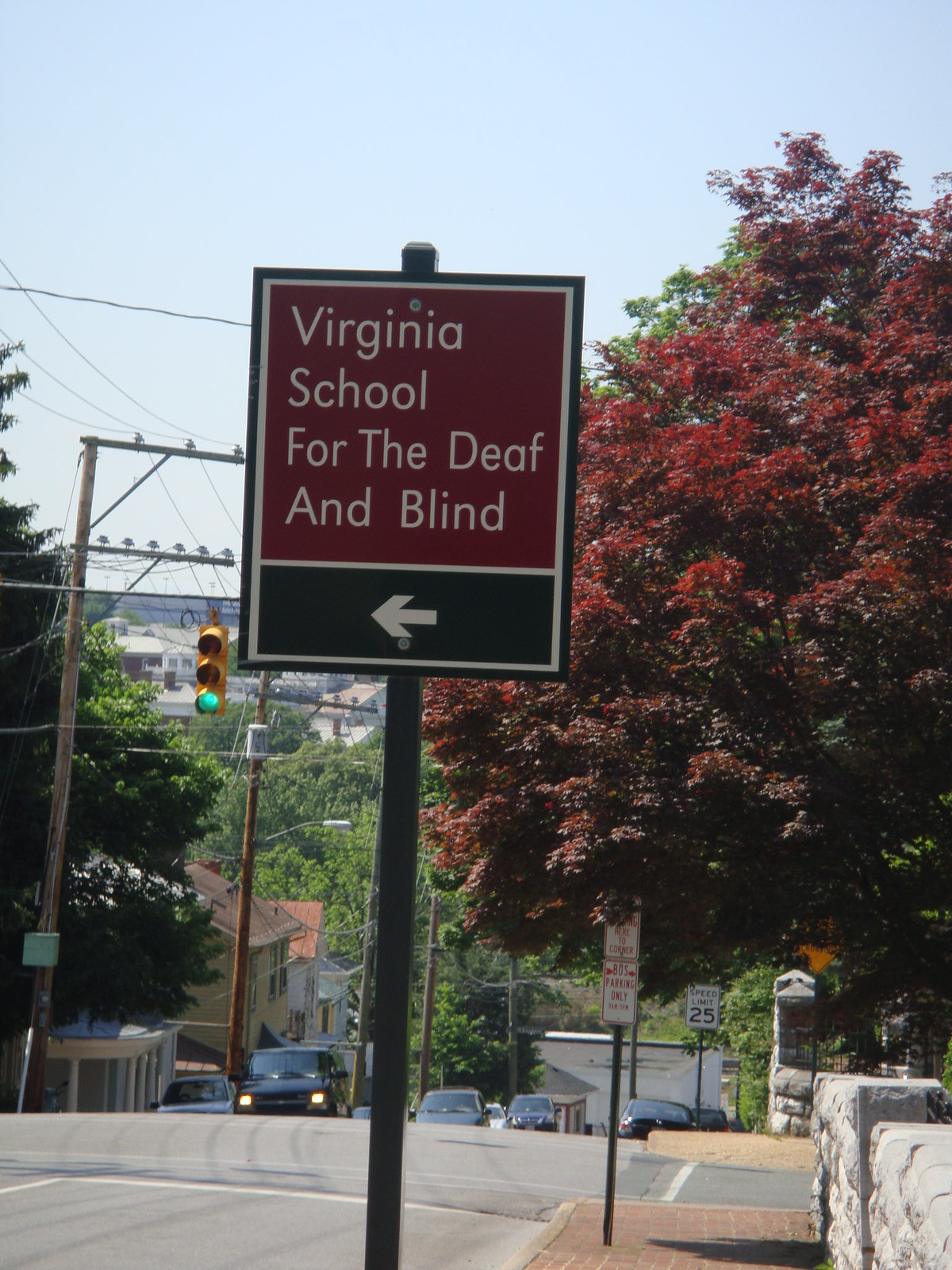This photograph captures a detailed street sign that stands prominently in the top half of the image, positioned at the center. The sign itself is large and square, bordered by a thin white line. The top three-quarters of its background are a muted red, not overly bright, while the bottom quarter is black. Displayed in white text, the sign reads: "Virginia," followed by "School," "For the Deaf," and "And Blind." A horizontal white line separates this text from a filled-in arrow at the bottom, which points to the left.

The sign is mounted on a black pole visible both below it and at the top center. The signpost is situated on the side of a road. To the left of the image, part of the street is visible. On the right side, a large, round tree with a mixture of green and red leaves stands out vividly against a light blue sky. Additionally, a green streetlight can be seen to the left of the sign, positioned almost directly below it.